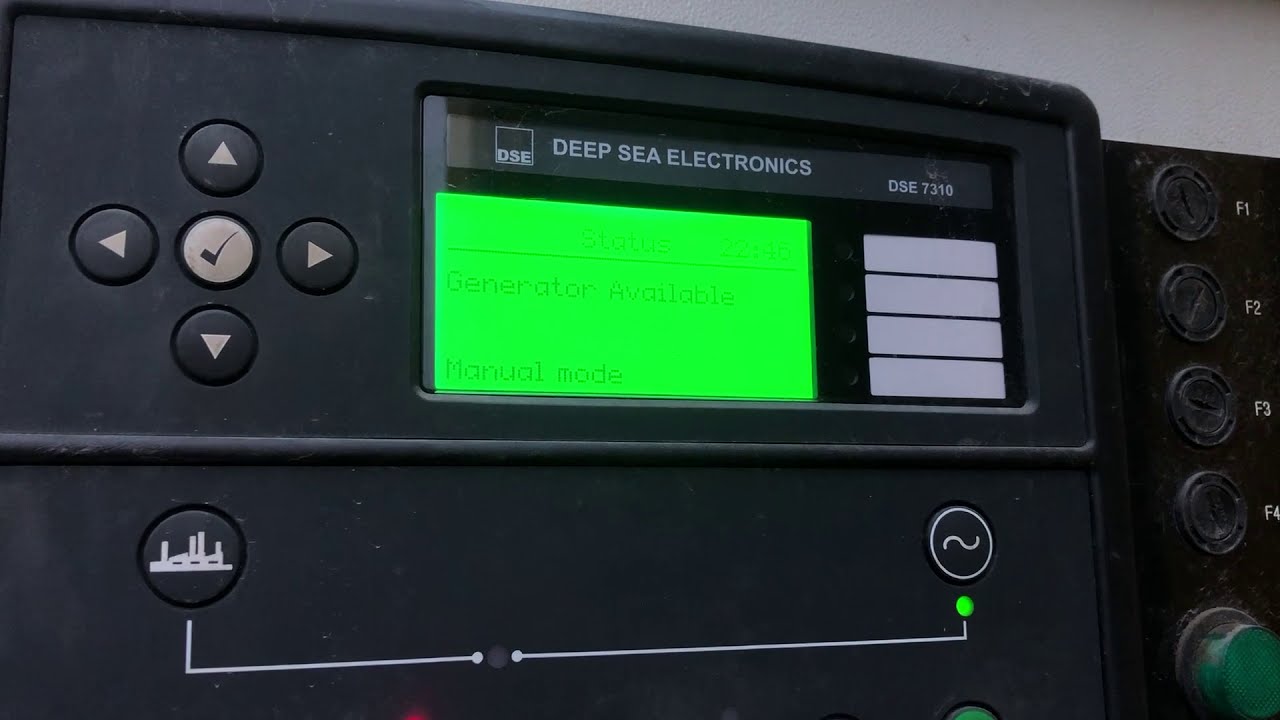The image depicts an up-close view of a black control panel for what appears to be a marine or oceanic instrument. Dominating the center of the panel is a bright neon green screen displaying detailed information. Above the screen, the name "Deep Sea Electronics" is prominently displayed, alongside the model number "DSE7310." The panel is covered in various buttons and knobs: to the left, there are directional knobs with arrows pointing up, down, left, and right; to the right, additional black buttons are situated; and at the bottom, there are further controls including black and white knobs and ports labeled F1, F2, F3, and F4. Texts present on the panel include "Generator Available" and "Manual Mode," which contribute to understanding its functionality. The panel is primarily black, with white, gray, and green details, and it occupies almost the entire image frame, indicating that this is an up-close photograph of the device.